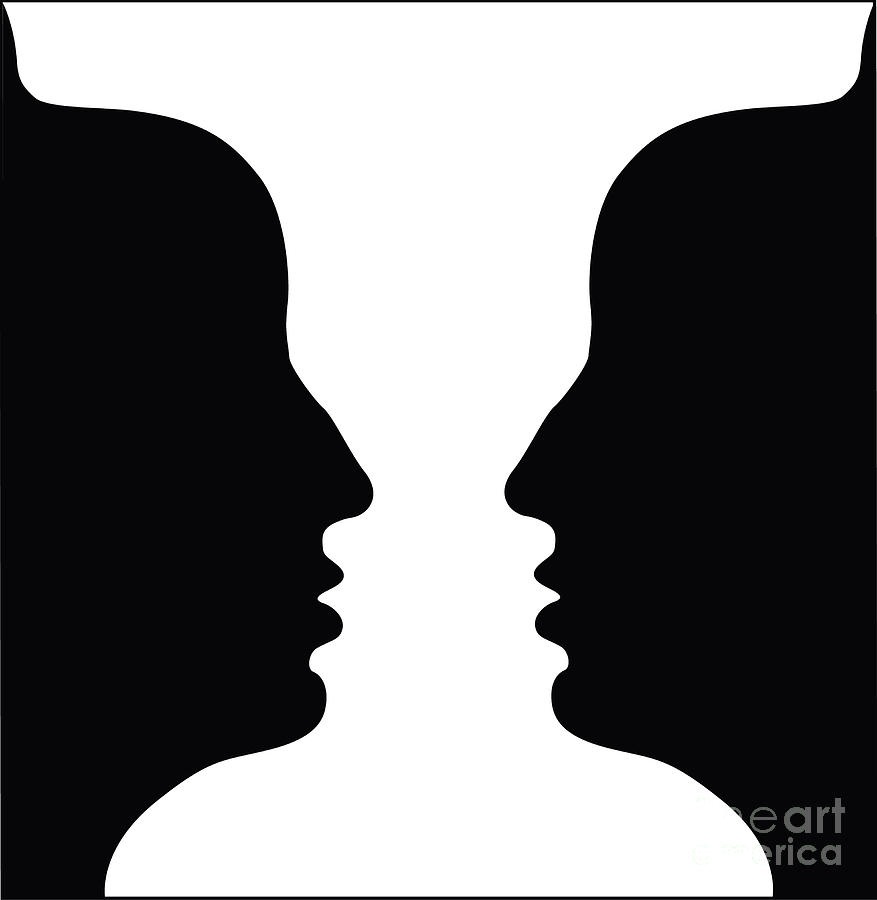This image is an intricately detailed optical illusion artwork, rectangular in shape and oriented vertically, with its height twice as long as its width. A thin black border outlines the top and bottom edges, while the left and right sides are likely obscured by the drawing itself. The centerpiece of the image features the shadowy silhouettes of two faces confronting each other; the face on the left is directed rightward, and the face on the right is directed leftward. These silhouettes include detailed features such as foreheads, noses, lips, and chins, though they notably sport batman-ear or horn-like points on top of their heads. Between the two silhouettes, the negative space forms a white candlestick or chalice, lending a dual interpretation to the artwork—viewers can see either the faces or the chalice. In the bottom right corner, there is semi-transparent gray text that reads "Fine Art America," adding a subtle yet identifiable watermark.